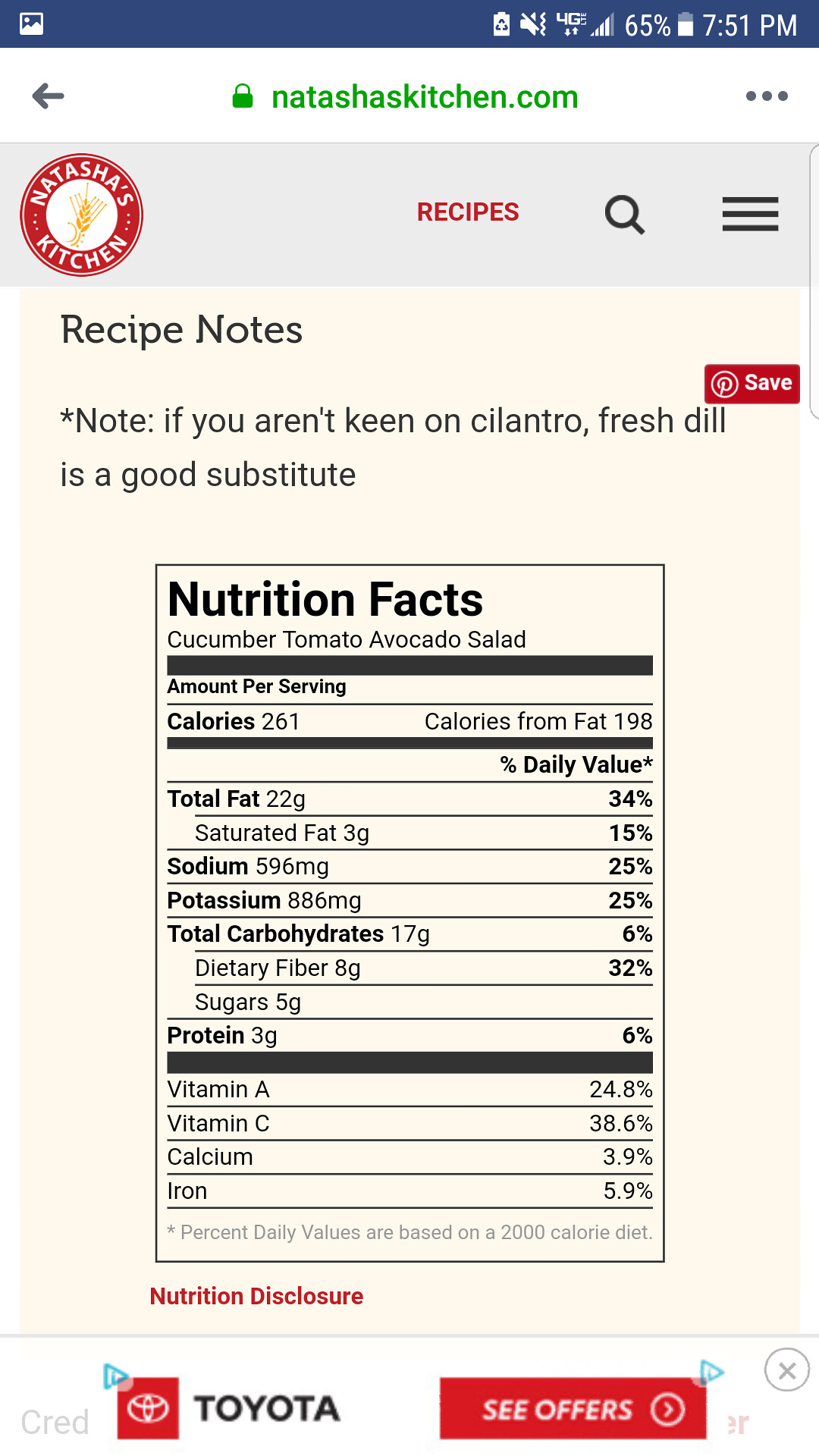A detailed screen grab of a nutrition label photographed on a mobile device, captured at 7:51 PM with a battery life of 65% visible at the top. The screen shows a webpage from natashaskitchen.com, featuring a recipe with accompanying notes. One tip advises that fresh dill can be a good substitute for cilantro. Below the notes, there’s an option to save the recipe to Pinterest. The nutrition facts provided are for a cucumber tomato avocado salad. At the bottom of the screen, there is an advertisement for Toyota, complete with a button to view offers and an 'X' to close the ad if preferred.